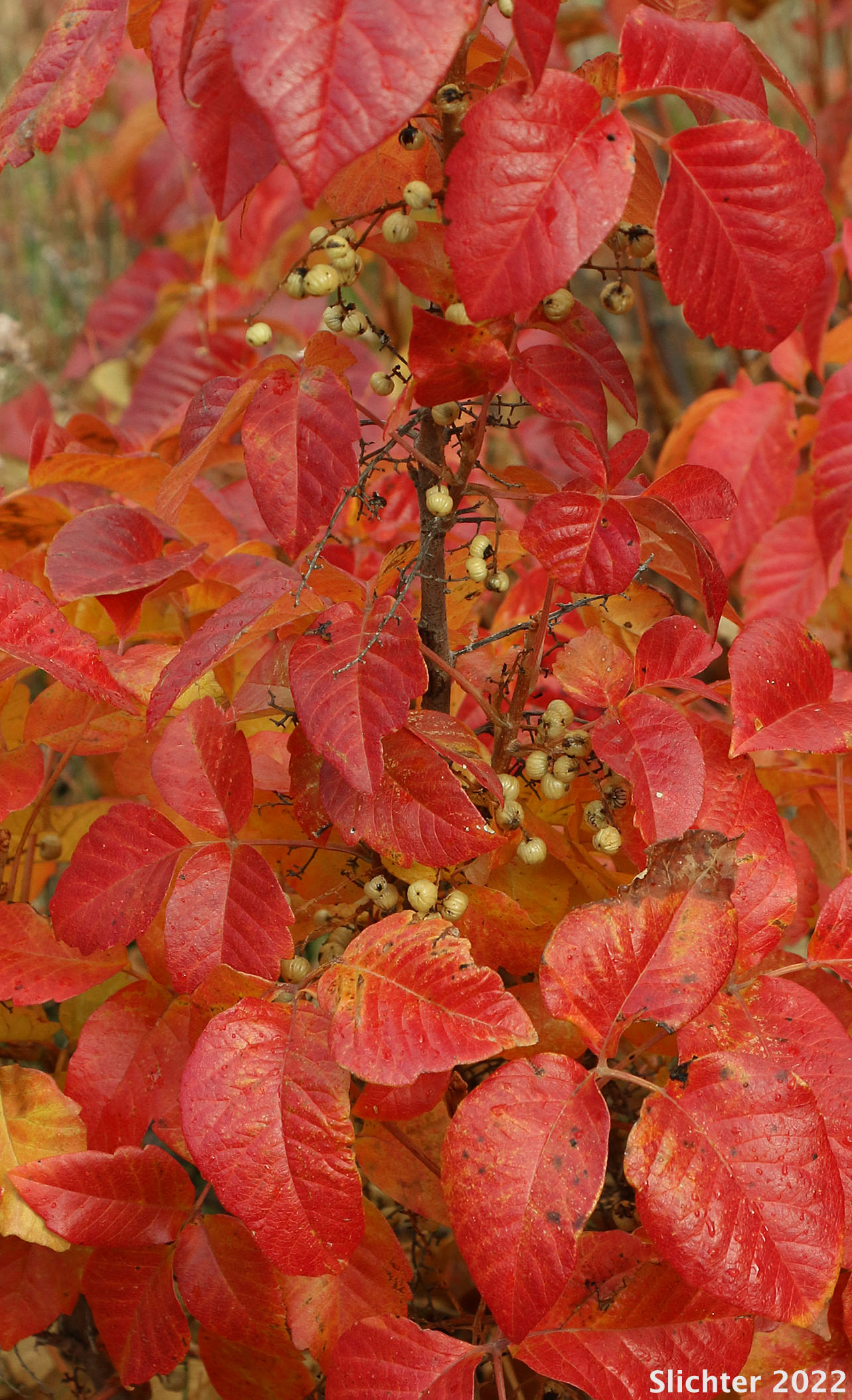This captivating photograph, titled "Slichter 2022," offers a close-up view of autumn foliage, featuring predominantly red leaves accented by tones of golden yellow and orange. The leaves are wider at the base, tapering to a point, and exhibit clear striations and veins, with some showing black and brown spots indicative of fading or insect activity. Interspersed among the leaves are clusters of small white berries, adding an additional layer of detail to the composition. The image captures a branch of the tree from which these colorful leaves stem, surrounded by sporadic small twigs and branches. The blurred background reveals hints of a grassy patch or wooded area, enhancing the natural autumnal feel. A subtle sheen on a few leaves suggests the presence of morning dew. In the lower right corner, the photographer's stamp, "Slichter 2022," is visible in white, marking the image with a personal touch.